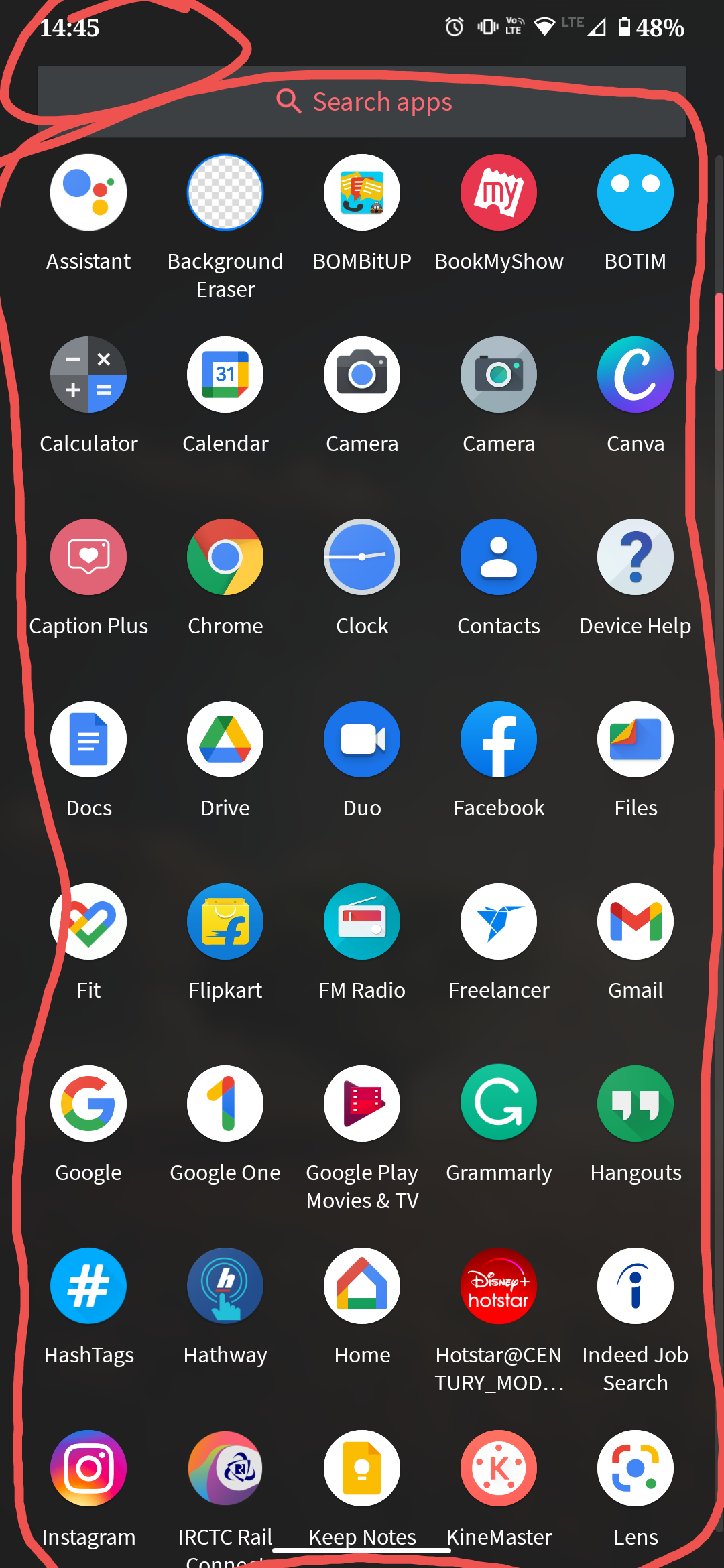The image is a screenshot from a smartphone displaying a variety of apps. In the upper left-hand corner, the time is shown as 14:45, highlighted with a red circle around it. Positioned near the top center of the screenshot is a search bar with the text "search apps" in red, which is also enclosed with a red outline extending down both sides of the screenshot, encapsulating the array of apps shown. The screenshot features a comprehensive list of apps neatly organized into rows. In the circled area, the apps listed are as follows: 
- First row: Assistant, Background Eraser, Bomb It Up, Book My Show, BOTIM, Calculator, Calendar, Camera, Camera
- Second row: Canva, Caption, Caption Plus, Chrome, Clock, Contacts, Device Help, Docs, Drive, Duo
- Third row: Facebook, Files, Fit, Flipkart, FM Radio, Freelancer, Gmail, Google, Google One, Google Play Movies & TV
- Fourth row: Grammarly, Hangouts, Hashtags, Hathway, Home, Hotstar, ICICI, Mod, Indeed Job Search
- Fifth row: Instagram, IRCTC Rail, Keep Notes, Kinemaster, Lens

The detailed view provides an insight into the user's app ecosystem, reflecting a diverse range of utilities and entertainment options.